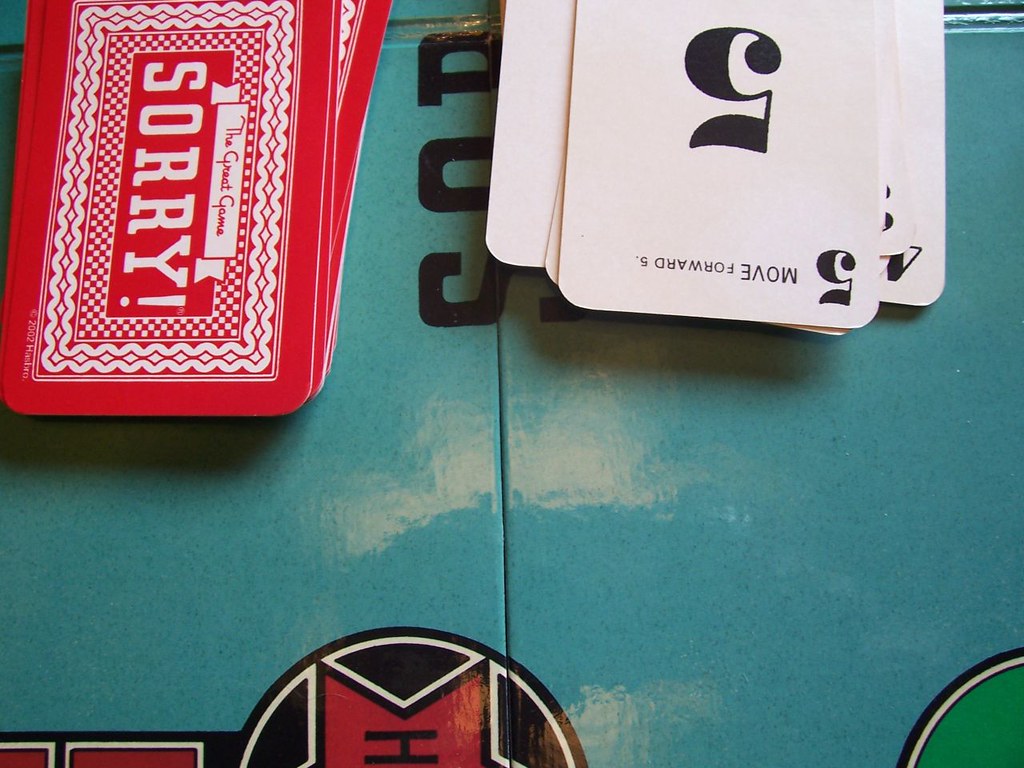The image showcases a vibrant game board prominently displayed on a turquoise blue background that takes up the entire frame. At the center, the partial view of the game board presents some letters that appear to spell "SOD" or "COD", though it is not entirely legible due to the board being cut off. Flanking the center are two decks of cards, one on the left and another on the right.

On the far right corner, a small green area is visible, delineated with white and black outlines, yet it is partially cut off. Moving toward the middle, there is an observed circle, also cut off, outlined in black and white. A red double triangle occupies the center, accentuated with black lines and bordered by white and black edges.

On the left side of the board, there is a black rectangular box containing two smaller dark brown boxes, both outlined in white and black. At the top left, several red playing cards are scattered with prominent white writing. One of these cards showcases "The Great Game" in a white box with red writing, and another card displays "Sorry!" in a red box with white writing, punctuated by an exclamation mark. These cards are accented with red and white checkered borders, along with wavy red and white designs, with the remaining card area also being red.

On the right side of the image, some cards are turned face-up. The top card prominently displays a large black number five at the top left corner, a large five in the center, and the instruction "Move forward to the five."